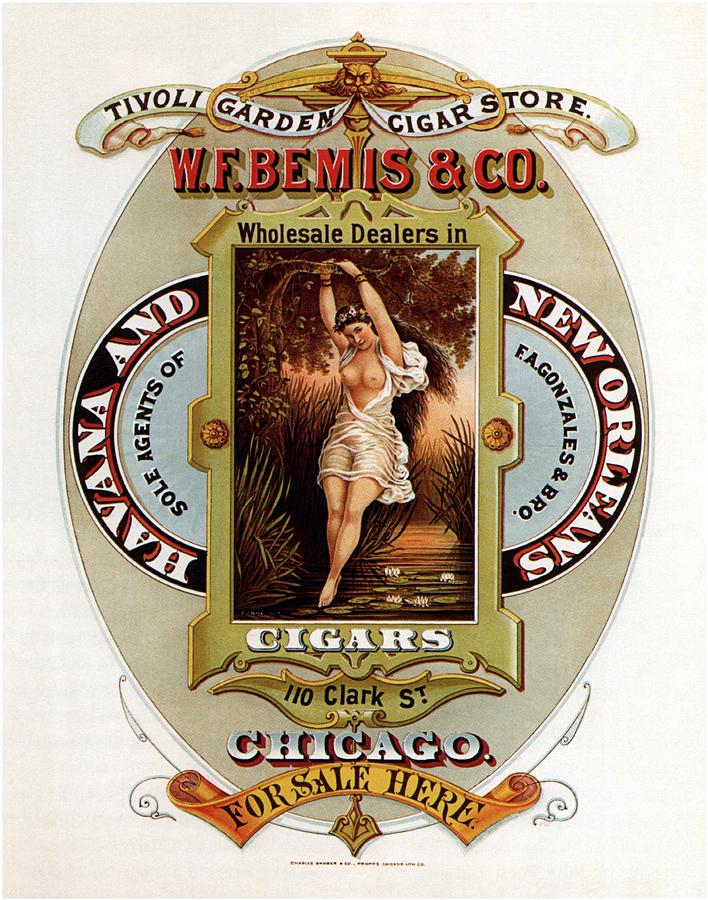This is a vintage advertisement for the Tivoli Garden Cigar Store. The ad is oval-shaped, filled with a light tan, parchment-colored background, and features intricate detailing. At the very top, there is a white ribbon bearing the store's name, "Tivoli Garden Cigar Store," followed by the red inscription "WF Bemis & Co." Below this, a light green rectangle with the words "Wholesale Dealers in Cigars" stands out prominently. The ad includes the location 110 Clark Street, Chicago, with "For Sale Here" noted at the bottom.

On the sides, the text denotes "Havana" and "New Orleans," highlighting them as the sole agents of F.A. Gonzales & Breaux. The central artwork features a painted woman with long, wavy dark brown hair decorated possibly with a flower crown. She is partially clothed in billowing white robes that leave her chest exposed. The woman is depicted standing barefoot above a pond adorned with lily pads, her hands bound above her head to a tree branch, adding to the dramatic and eye-catching imagery.